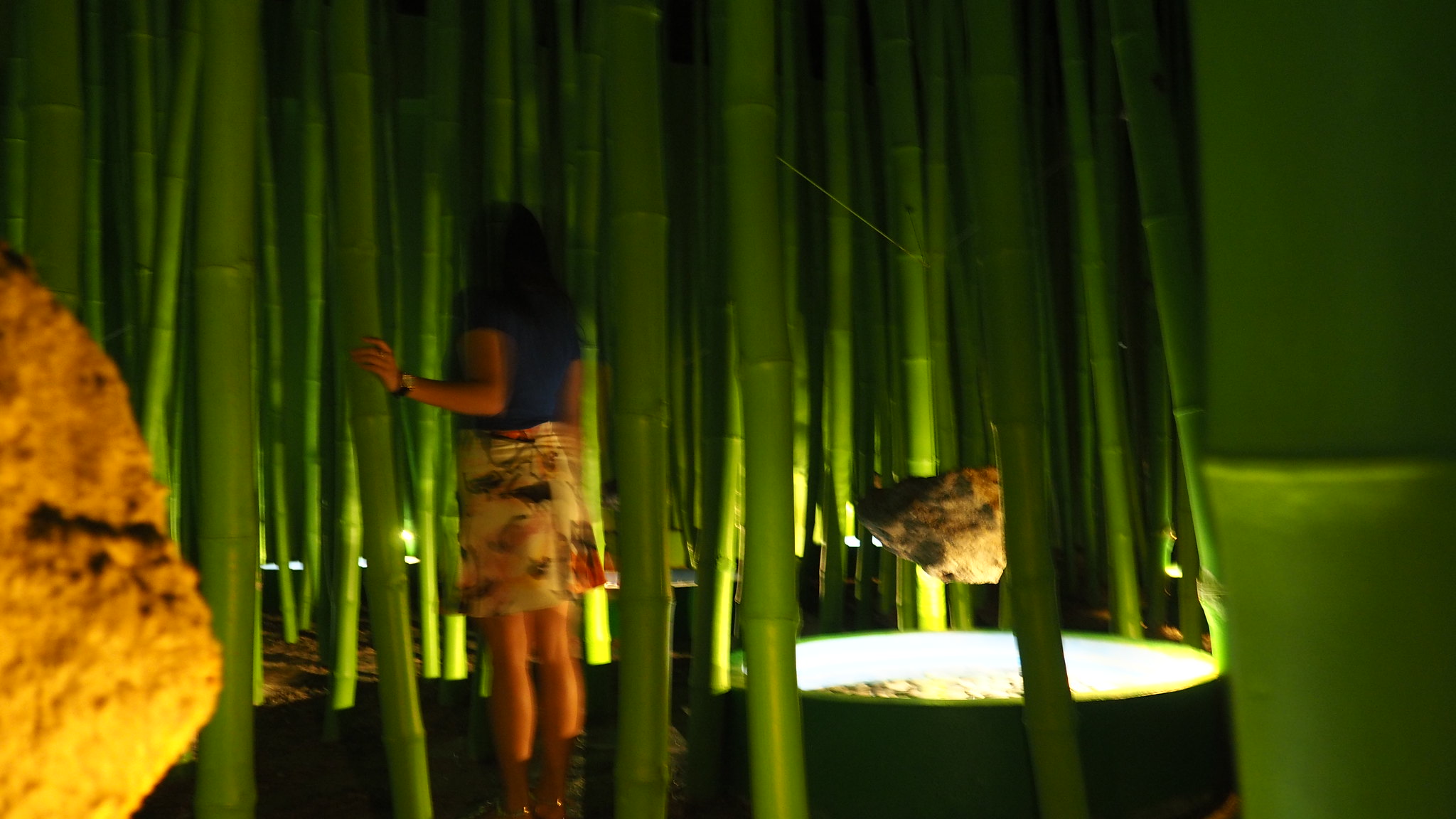In the center of the image stands a girl with long, dark brown hair cascading down her back, reaching between her shoulder blades. She wears a navy blue short-sleeve blouse paired with a white skirt adorned with colorful bug designs, which falls above her knees, leaving her legs bare. She is set against a backdrop that appears to be a bamboo forest, though the bright green bamboo stalks have a somewhat plasticky texture and are hanging from the ceiling. The setting is well-lit by a large, oval, bright white light on the lower right side of the image. This light illuminates a brown rock, which appears to be suspended or floating above a circular pool of light. Additionally, there is another similar rock with a meteorite-like texture positioned on the floor, adding to the unique atmosphere of the scene. Her left arm holds onto one of the bamboo stalks, grounding her in this whimsical environment.